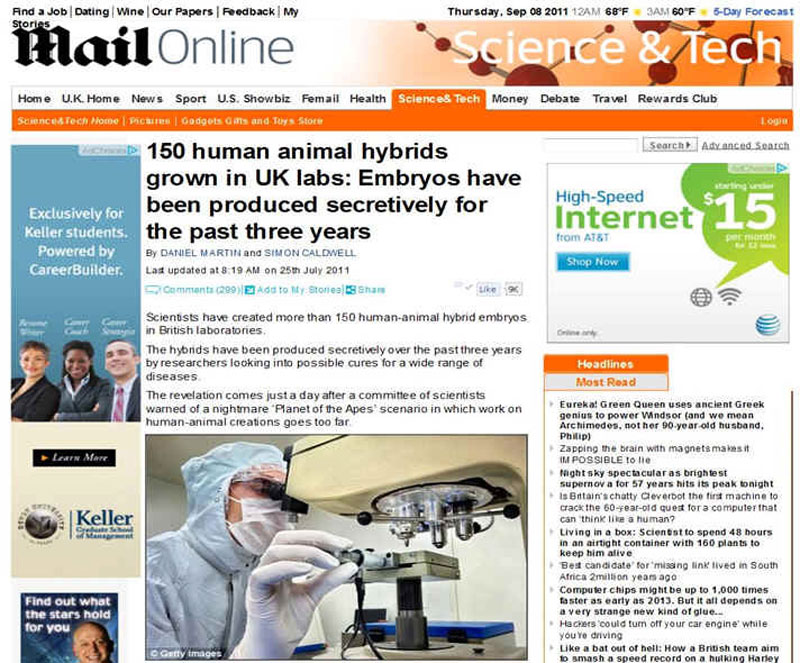The image depicts an online meal publication from Thursday, September 8th, 2011. At the top of the page, a series of navigational headings are displayed: Home, UK Home, News, Sport, US Showbiz, Female, Health, Science and Tech, Money, Debate, Travel, and Rewards Club. The section currently selected is “Science and Tech,” featured prominently as the front page splash.

Dominating the center of the page is a controversial headline: "150 human-animal hybrids grown in UK labs. Embryos have been produced secretly for the past three years." This article, dated July 25th, 2011, reports that scientists have created over 150 human-animal hybrid embryos in British laboratories, sparking ethical debates.

To the left of the main story, there are three advertisements. The first promotes Career Builder, targeting Keller students exclusively. The second is an advertisement for Keller, which appears to be a management firm. The third ad is a horoscope-related piece, enticing readers with insights about their astrological fortunes.